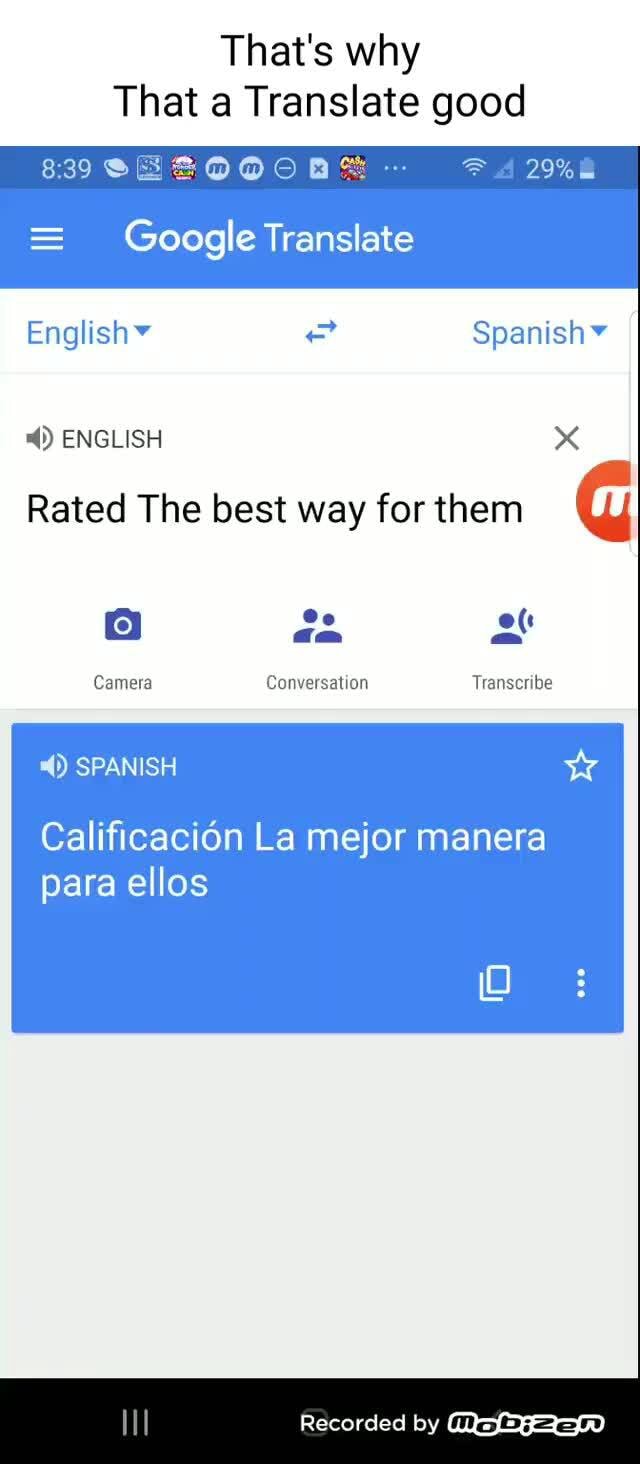The top portion of the image features the phrase "That's why I translate good," which appears to be displayed prominently. The image itself seems to be a screenshot from a mobile phone, as indicated by its portrait orientation. In the upper left corner, you can see the time along with various icons: a Wi-Fi symbol, an unidentified icon, and a battery icon indicating a 29% charge.

A well-illuminated bar appears at the bottom, contrasting with the overall shaded background. The primary content showcases the Google Translate app, identifiable by the app's logo in the upper left corner alongside three horizontal lines, commonly known as the menu icon. Below this, "English" is displayed with a downward arrow, suggesting a dropdown menu for selecting languages.

In the center are two horizontal arrows pointing left and right, likely for swapping the "from" and "to" languages. On the right side, "Spanish" is accompanied by a downward arrow, indicating the selected target language.

The main body of the screenshot displays the translated text, reading "The best way for them," written in English. Beneath this text, there are several icons for different functionalities. These include a camera symbol labeled "Camera," a vector icon of two people labeled "Conversation," and another icon of a person with radiating curves labeled "Transcribe."

Below this section, a blue text box appears with the Spanish translation: "Calificación lava amendra para ellos." Various interactive symbols lie at the bottom of the screen, indicating additional functionalities.

At the very bottom of the image, a label reads "Recorded by Mosin," suggesting that this screenshot was captured using a screen recording tool by the named user.